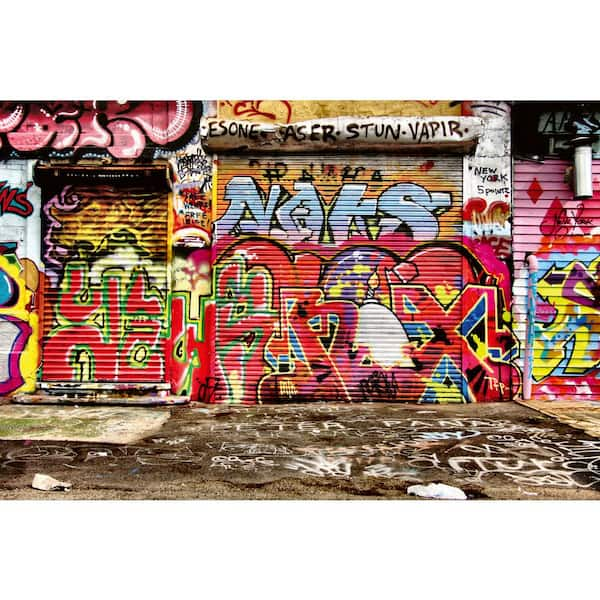This photograph captures a gritty urban scene featuring a row of narrow garage-type buildings, commonly used by city vendors to sell their goods. Each building's metal pull-down door is closed and extensively adorned with high-quality, vibrant graffiti, creating a visually striking tableau. The graffiti showcases an array of overlapping symbols, shapes, and letters, with colors predominantly including red, pink, and various other hues. Despite the abundance of intricate details, the clearly readable letters across the doors spell out "N-O-K-S," "E-S-O-N-E," "S-T-U-N," and "V-A-P-I-R." The rightmost door has a pink background, while the leftmost appears to have flame-like designs. Below the garages, the dirty cement ground is marked with white-painted graffiti and uncleaned algae, completing the picture of an urban space where art meets decay.